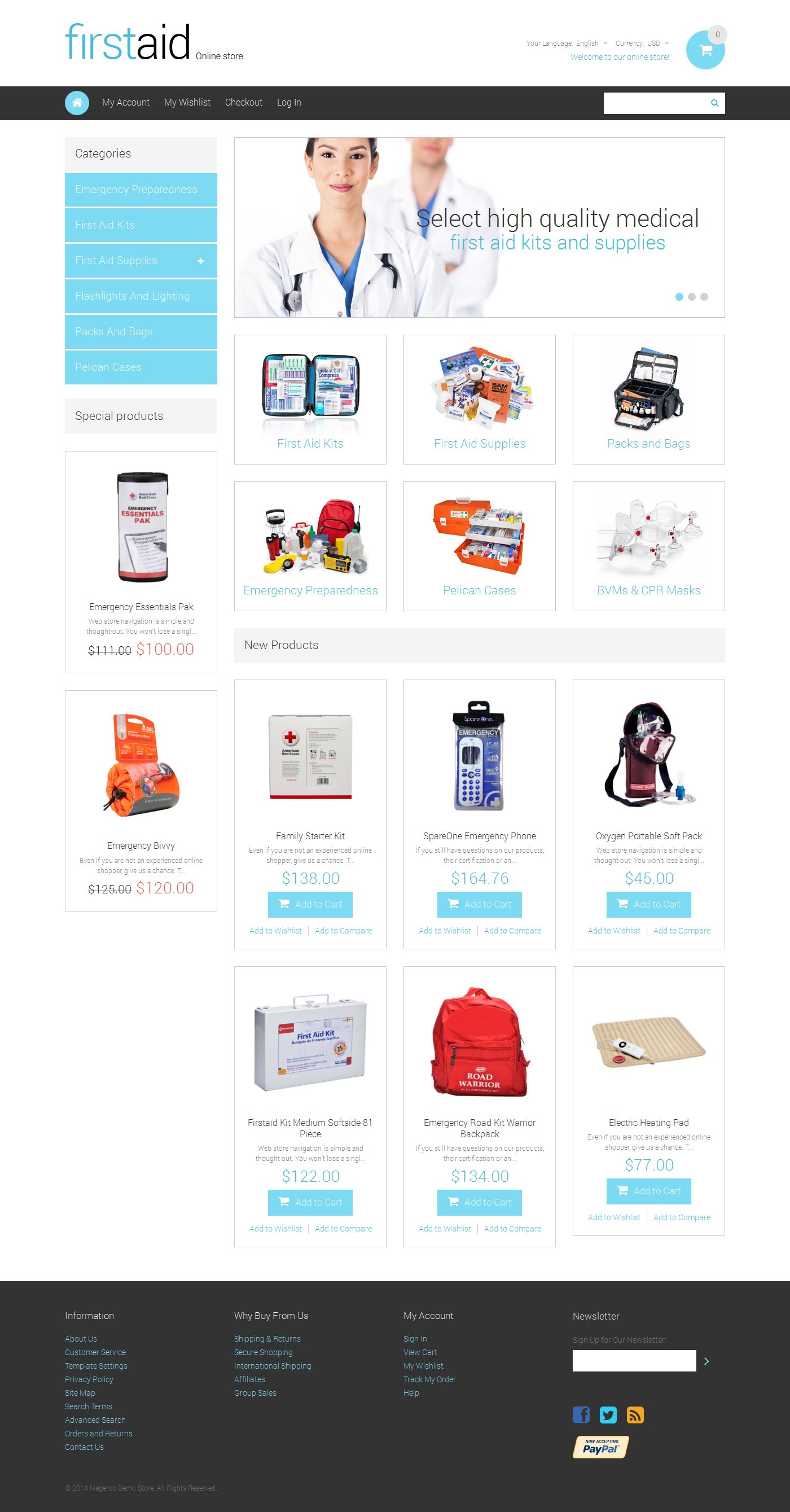Top right corner displays "First Day" and "Online Store." There's an option to select language displayed as "Your Language / English" and currency set to "USD." Navigation elements include a blue circle with a shopping cart icon, a welcome message to the online store, and a grey circle on the top right.

A black bar at the top of the page contains icons for "My Account," "My Wishlist," "Checkout," and "Login," all placed within a white navigation bar. The sidebar features a list of categories in light blue squares, including "Emergency Preparedness," "First Aid Kits," "First Aid Supplies," "Flashlights and Lighting," "Packs and Bags," and "Pelican Cases."

Above these categories, there's a section labeled "Special Products." The top of this section highlights "Select High-Quality Medical First Aid Kits." The products listed include:

- Emergency Essentials Pack: $111 and $100
- Emergency Preparedness Pelican Cases, PVMs, and CPR Masks
- Emergency Family Starter Kit: $138
- Spare One Emergency Phone: $164.76
- Blue XR Oxygen Portable Soft Bag: $45
- First Aid Kit: Medians Outside 81p: $720
- Emergency Real Kit Warrior Backpack: $134
- Electric Heating Pads: $77